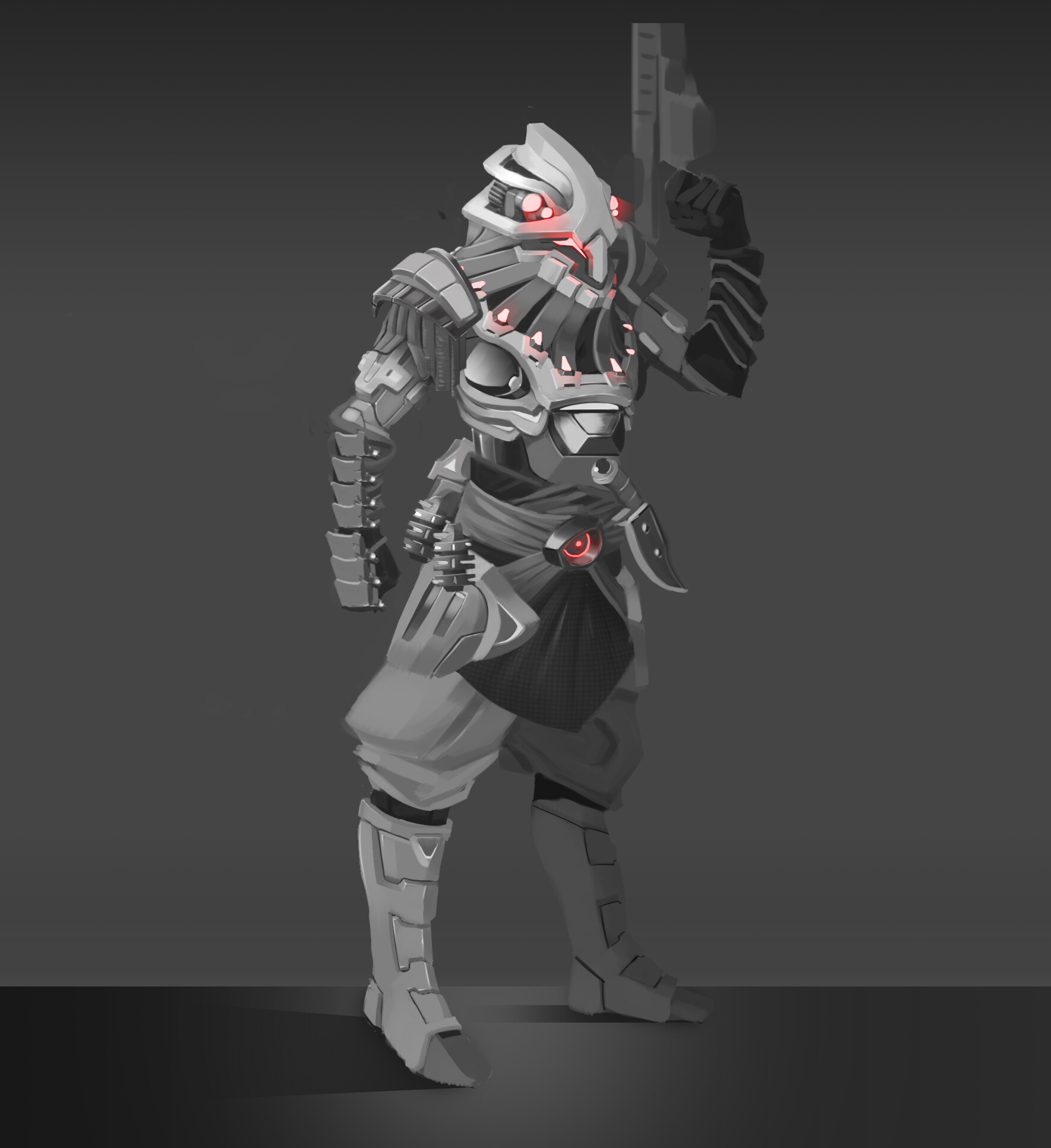This intricate artist’s drawing features a robotic fantasy character standing against a dark gray background, with a near-black floor beneath it. The robot's design is highly detailed and blends futuristic elements with historical notes. The robot has a head equipped with four glowing red eyes, arranged in pairs with two large ones and two smaller, indented ones, resembling headlights. Covering its face is a shield-like helmet, reminiscent of the Facehugger from the Alien movies. 

Its neck is adorned with what looks like dreadlocks or fringe, each strand featuring small red glowing triangles. This robotic figure appears armored, with individual rivet-style brackets running down its forearms. The robot wears a belt buckle that glows red and has a knife in a case hooked just above the belt. Attached to the belt are two spiky, pineapple-style grenades.

The robot has one gray leg and one black leg, dressed in what appears to be pantaloons, a historical style that bulges at the thighs and narrows down to individual metal plates forming boots. In its left hand, raised beside its head, it holds a large, handgun-like weapon. This weapon is gray and appears short yet thick, suggesting it’s a stubby but formidable firearm. The right arm hangs down to its side, not holding any weapon. The overall design gives a sense of a fearsome, battle-ready mechanical entity standing sentinel in its dark environment.